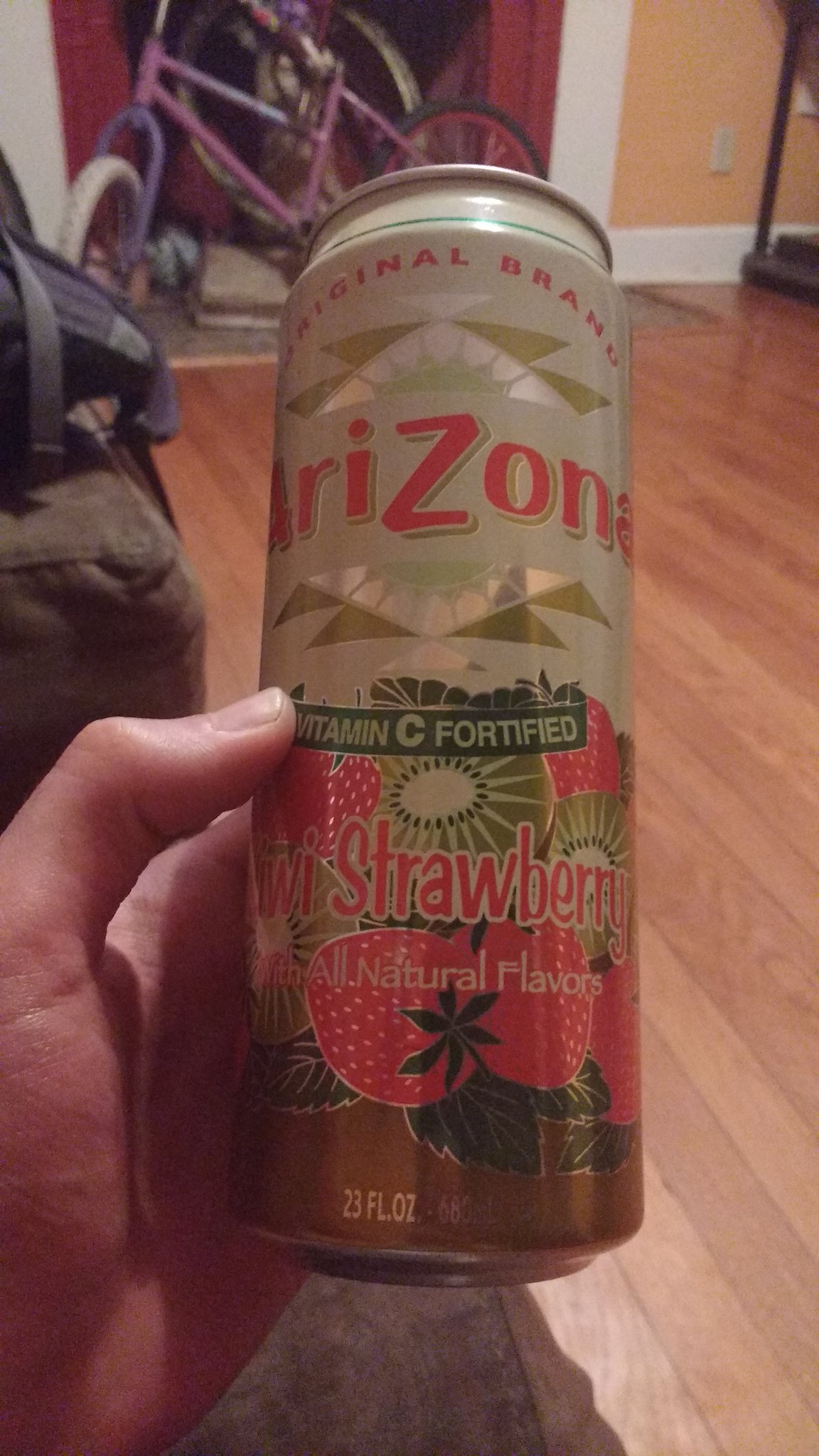In a typical household room with medium-toned wooden maple flooring, a photograph captures a close-up view of a left hand holding a can of Arizona Kiwi Strawberry juice drink. The hand is coming up from the bottom left corner, wrapping its thumb around the left side of the can, which is held at a slight slant. The can's design features a tan, almost off-white background with gold highlights and geometric patterns. Bold red and coral lettering spell out "Arizona" across the top half, with a green banner underneath proclaiming "Vitamin C Fortified." Below this, detailed illustrations of whole strawberries, kiwi slices, and green leaves accompany the text "Kiwi Strawberry" in bright pink and "All Natural Flavors" in white. The can is marked as 23 fluid ounces. 

In the background, the room's pale apricot walls frame a scene of casual domesticity. On the extreme left side, the edge of a chair or brown couch is visible, cluttered with assorted items. The back of the room features a child's pink bicycle leaning against what might be a wall or closet door. There's also a small rug near the bicycle and a piece of art with a white border, dark pink inside, and black accents hanging on the upper left side. To the upper right, a piece of black exercise equipment or stand is partially visible, completing the room's homely yet busy atmosphere.